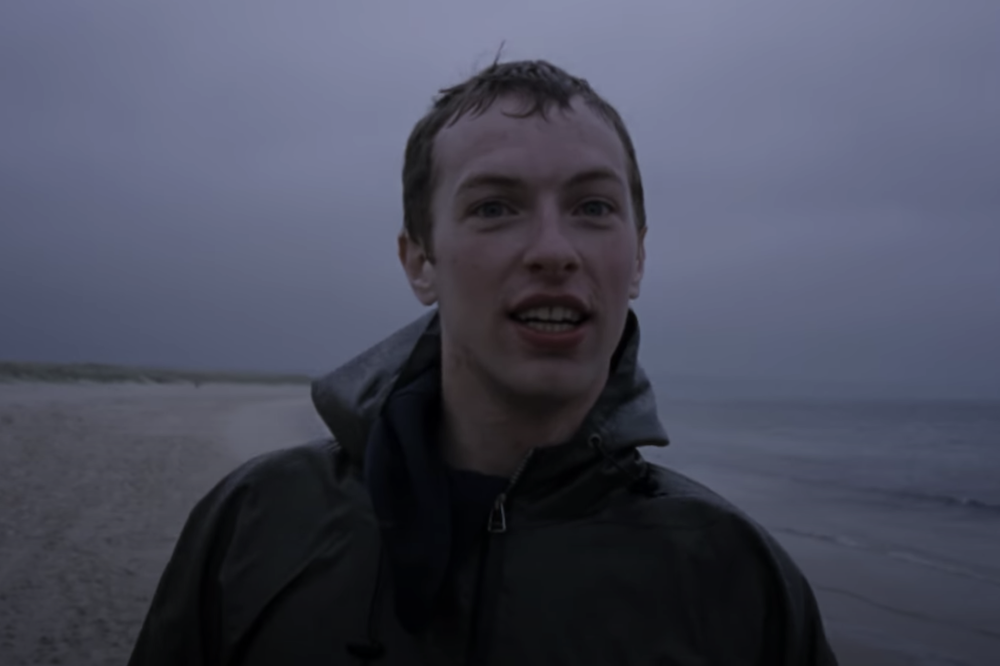The image is a detailed close-up photograph of Chris Martin from Coldplay, captured against a beach shoreline at twilight. Dominating the center of the frame, Chris stands on the wet sand with gentle waters lightly splashing nearby on the right side. His short, light brown hair appears wet, and he's attired in a dark green, almost khaki windbreaker-style rain jacket paired with a dark blue hoodie, though the hoodie is not worn up. Chris is looking directly at the camera, his mouth open as if caught mid-song, revealing his teeth. The setting is visibly dark and gloomy with heavy, overcast clouds looming above. On the left side of the photograph, there are patches of green grass adding contrast to the light-colored sand. The overall aesthetics suggest an early Coldplay era, likely around their debut album, characterized by Chris's youthful appearance and the moodiness of the environment.